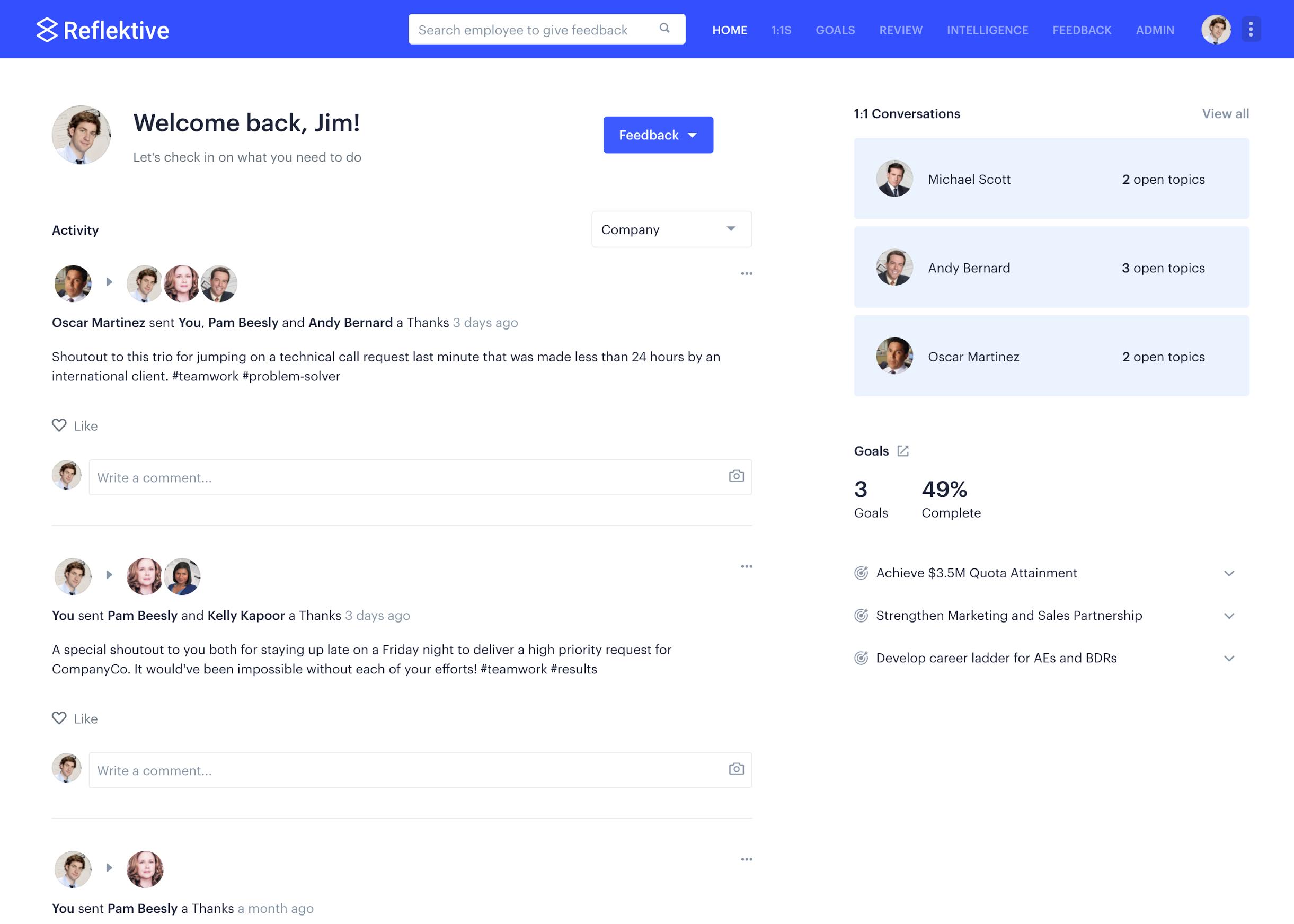The image showcases a screenshot of the website Reflectiv, spelled R-E-F-L-E-K-T-I-V. The logo, which features two stacked diamond shapes, is prominently displayed in white. Central to the website’s interface is a search bar accompanied by the phrase "Search employees to give feedback" and a magnifying glass icon. 

On the right side of the top navigation bar, several options are visible in white text: Home, 1 on 1, Goals, Review, Intelligence, Feedback, and Admin. Adjacent to these options is a circular profile picture of Jim Halpert from "The Office," along with the greeting "Welcome back, Jim."

The main section displays feedback activity, marked by a dropdown arrow next to the word "Feedback." Notably, the feedback section includes a satirical note where Oscar Martinez recently thanked Pam Beasley and Andy Bernard three days prior. The image also mentions several characters from "The Office," including Pam, Andy Bernard, and Oscar, alongside their interactions. 

To the right, a sidebar shows ongoing one-on-one conversations with Michael Scott, Andy Bernard, and Oscar Martinez. The goals section indicates that 49% of set goals have been completed, providing a quantitative measure of progress. The detailed layout and satirical references tie back to the humorous nature of the show "The Office."